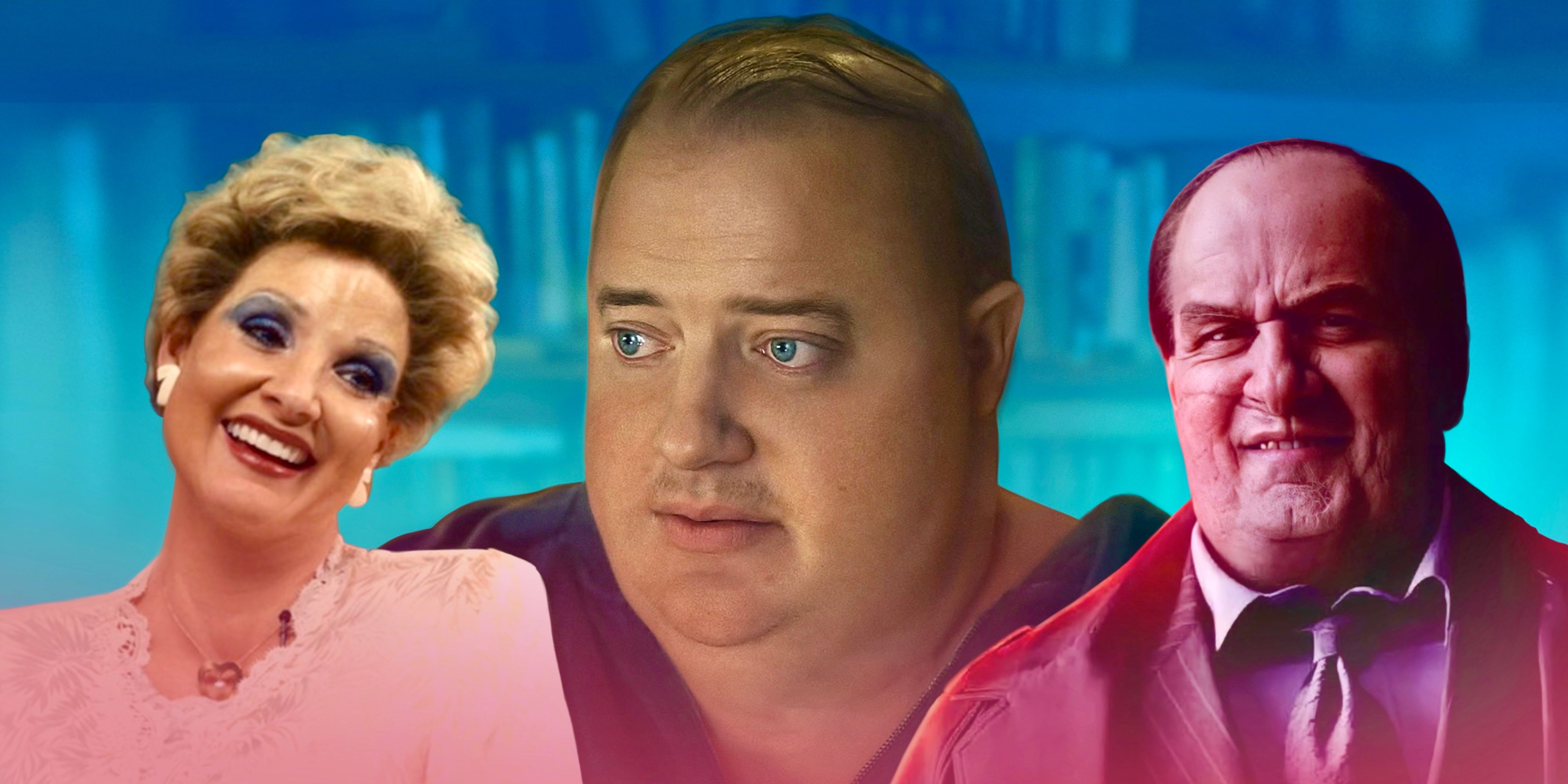This image, likely designed as a YouTube or video site thumbnail, features a heavily blurred and blue-tinted bookshelf background, giving it a distinct yet indistinct look. In the center stands Brendan Fraser, captured from his role in "The Whale," characterized by his overweight appearance, vivid blue eyes, and a V-neck t-shirt. On the left is a heavily made-up older woman with short, curled blonde hair, blue eyeshadow, bright lipstick, and white heart-shaped earrings, dressed in a pink top with lace around the collar and a necklace with a pink medallion. On the right, a classic movie villain figure, tinted red, appears as an older, clean-shaven man with a sinister grin, dressed in a suit and tie, reminiscent of the Penguin from an upcoming 2024 film.